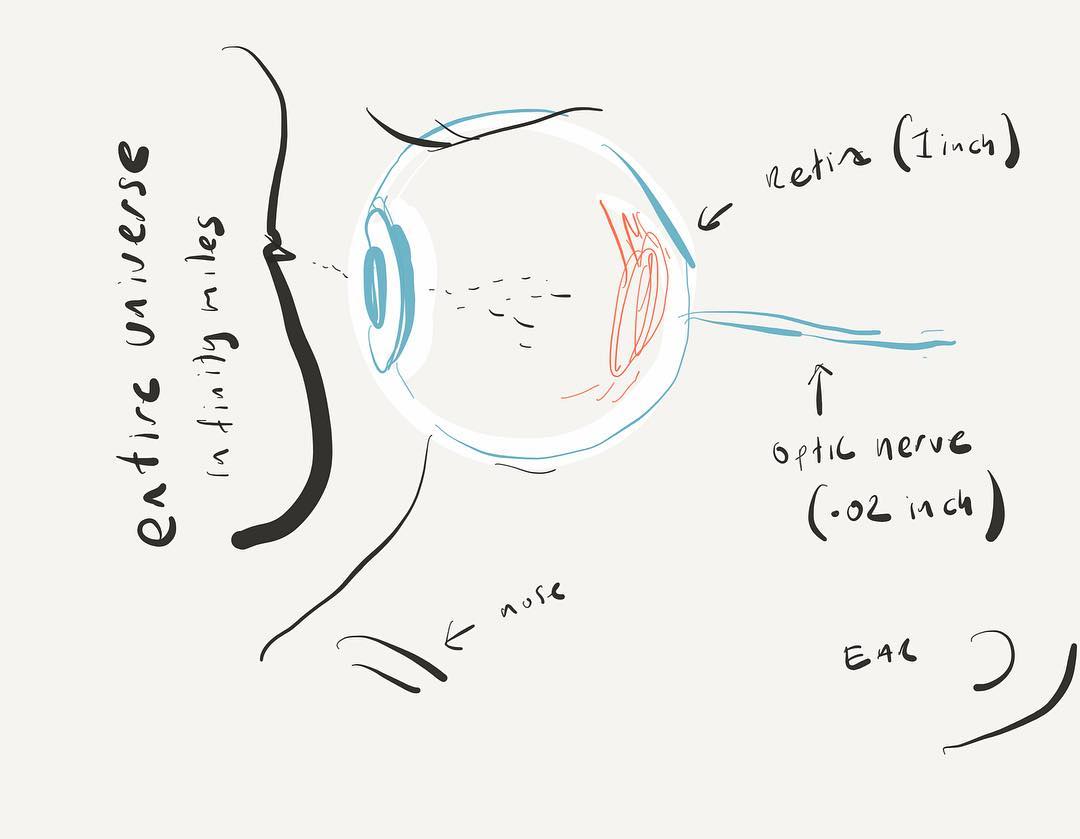This image is a detailed, hand-drawn sketch of an eyeball on a light gray background, complete with various labels and annotations. The eyeball is positioned slightly above the center and features a crudely drawn blue pupil and iris. The eyelid or eyelash is represented by a black line at the top of the eye. Inside the eye, towards the back, there are red squibbles that likely depict the retina. Behind the eye, a blue line symbolizes the optic nerve, annotated with "optic nerve, 0.02 inch."

To the top right of the eye, a yellow-orange section is labeled "retina, one inch" with an arrow pointing to it. In the largest handwritten text on the left side, it reads "entire universe infinity miles," with lines suggesting light entering the pupil. A vague outline of a nose is also indicated on the left, with an arrow labeled "nose." At the bottom, the word "ear" is written near a squiggly line representing an ear. This rough sketch serves as a labeled diagram highlighting various parts of an eyeball and their relative positions.